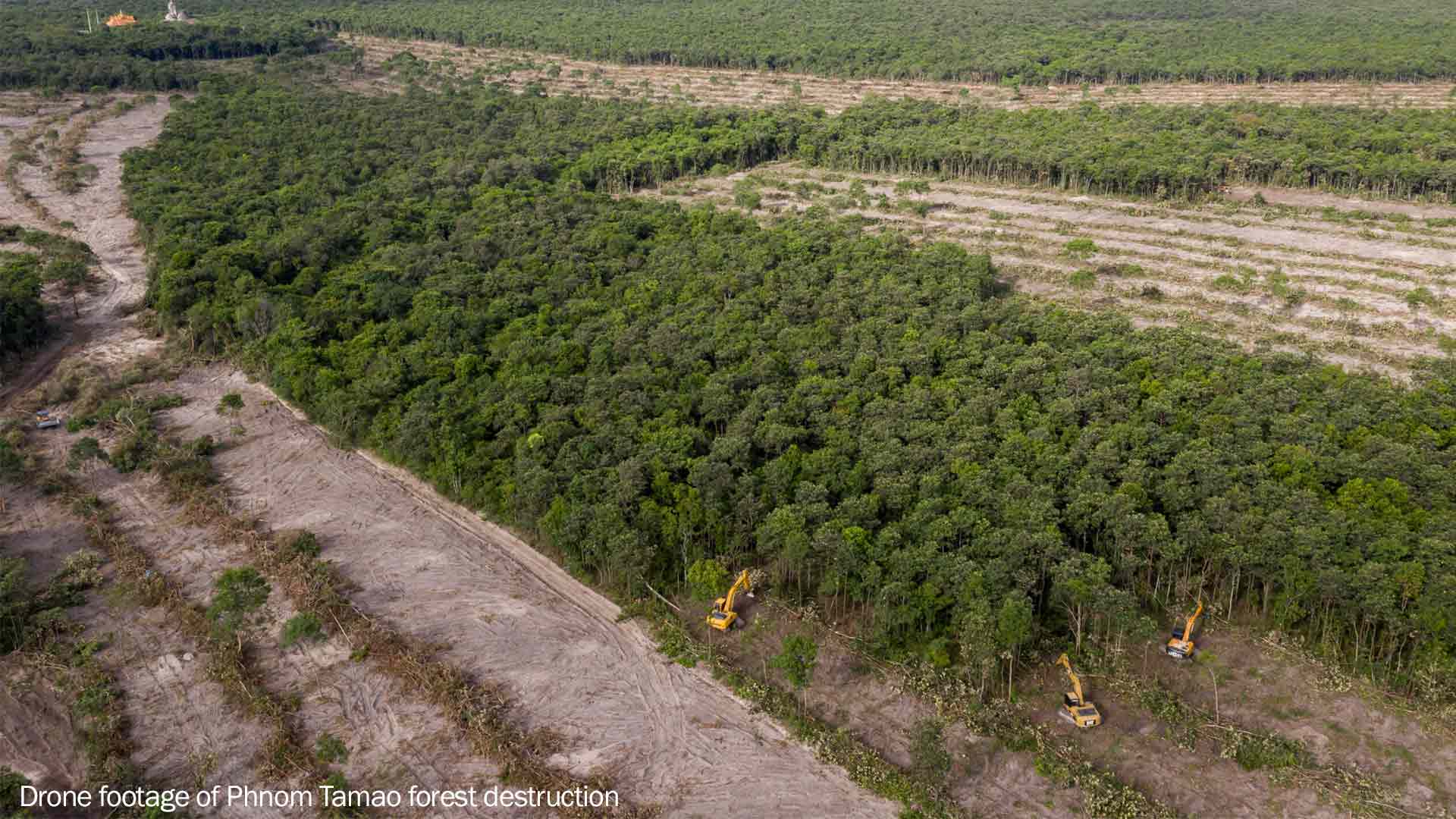This expansive overhead photograph captures the dramatic destruction of the Phnom Tamao forest in real time. In the center of the image, a dense, highly forested area is being aggressively cut down by three yellow bulldozers, which are clearly visible working in the foreground. Surrounding this central patch, vast swathes of land have already been cleared, revealing barren, sandy soil. Several roads and paths crisscross the landscape, marking the areas that have been stripped of trees. The top left of the image appears to serve as a base for the machinery and storage of the felled wood. The caption at the bottom of the photo reads, "Drone footage of Phnom Tamao forest destruction," underscoring the devastation captured in this horrifying scene.